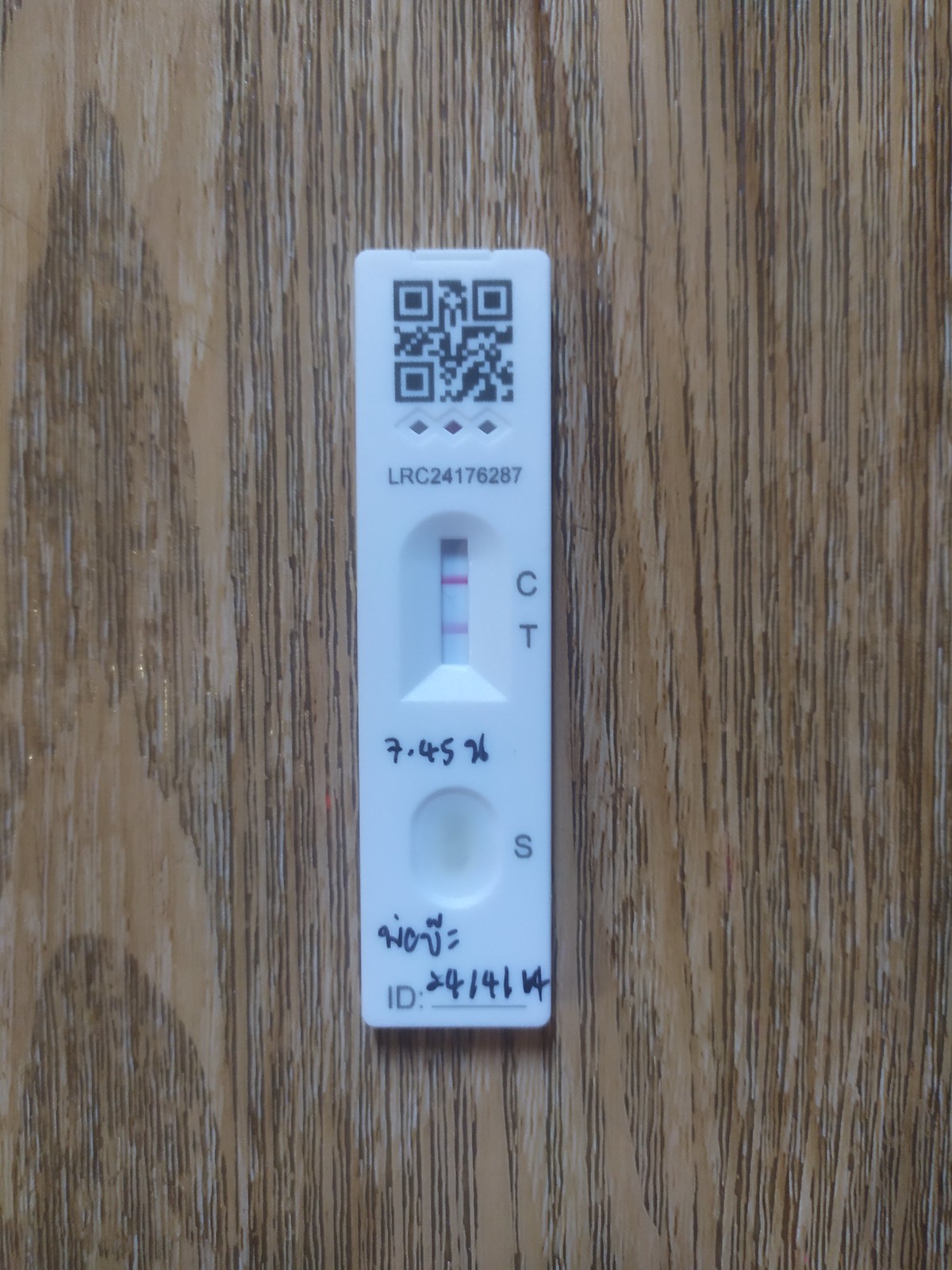The color photograph depicts a small, white, rectangular medical test strip placed on a wooden table surface with visible wood grain, suggesting a close-up shot. At the top of the test strip, there is a QR code followed by the identifier "LRC 24176287." Below this, there is a window for test results, resembling those found in pregnancy tests. The window is an arc-shaped depression containing a rectangular strip with three lines: a thick black line at the top, a red line labeled "C" on the right, and a pink line labeled "T" below it. 

To the right of the indicator window, "7.45%" is written in permanent marker, followed by an additional unrecognizable symbol. Below the main test window is another well marked with "S," which appears empty. Further down, more text is written in marker, but it is illegible. The bottom of the test strip features an "ID:" label, followed by a line and a partially visible ID code, seemingly "2414114," but the last digit is unclear.